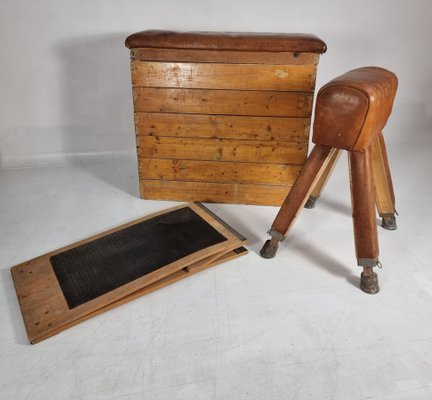In this photograph set in a room with a white floor, there are three prominent wooden objects. The first object, positioned at the center, is a sturdy stool with four black feet, featuring a smooth leather top, inviting one to sit or place items on it. Adjacent on its left is a unique rectangular wooden device with a black matte rectangular section in the middle, resembling a folded washboard. To the right of the stool stands a taller wooden structure resembling an ottoman but with additional height. This piece, made from stacked wood, boasts a cushioned seat and offers storage capability, indicating it can be used for seating, footrest, or storage. Each of these items shares the warm, natural brown tones of wood, enhancing their cohesive appearance in the room.